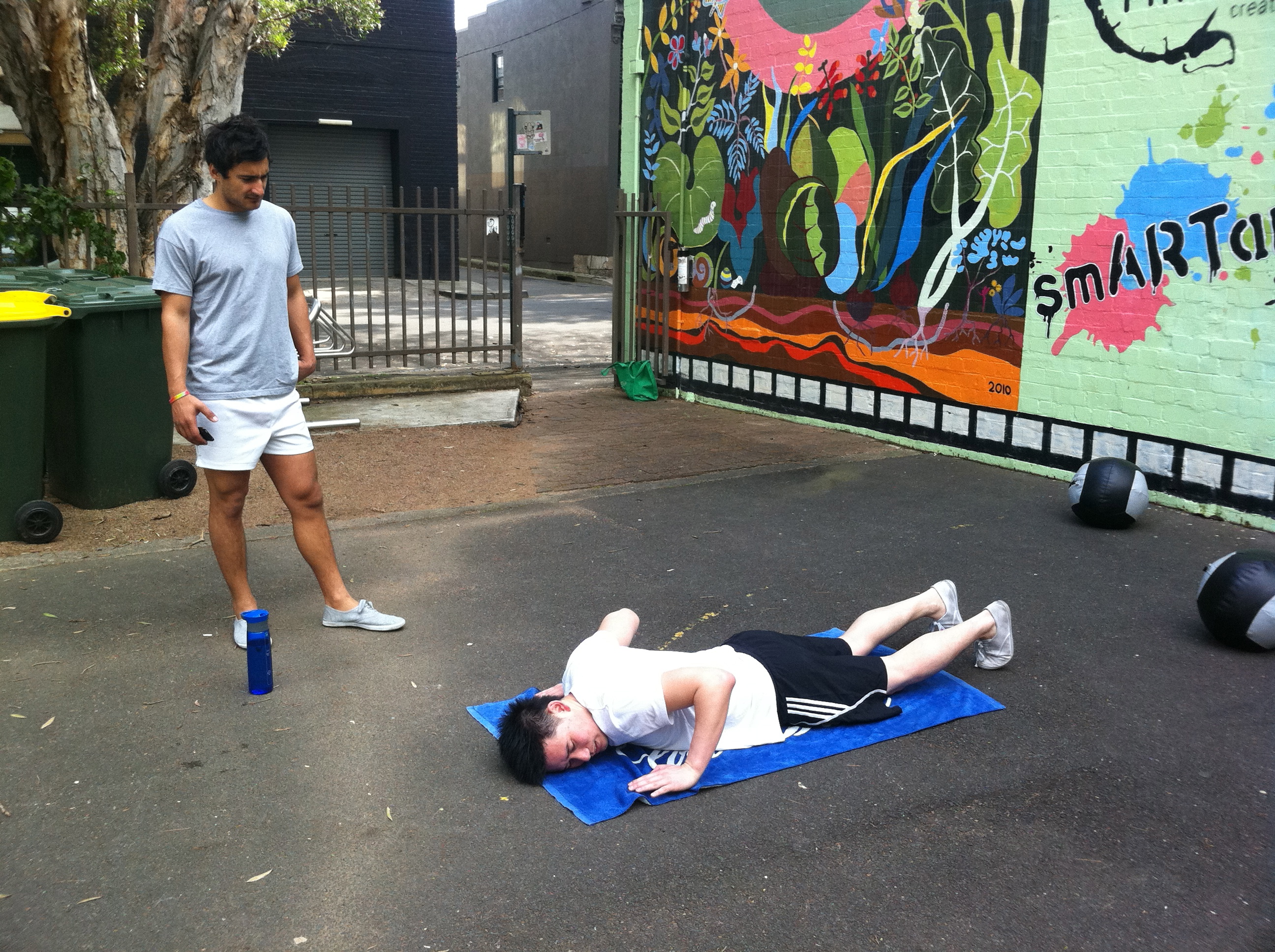The image depicts an outdoor scene during the day, featuring two men engaged in a workout in an urban setting. One man, who appears to be a coach, stands on the left. He is dressed in a gray t-shirt, white shorts, white sneakers, and a gold bracelet while holding a phone. Beside his foot is a blue water bottle. Behind him is a tree, a fence, and two green recycling bins, one with a yellow lid. In the center, another man lies on a blue towel on the blacktop, positioned as if about to do push-ups. He wears a white t-shirt, black Adidas shorts with white stripes, and white sneakers, and has black hair. Nearby, there are two black and gray medicine balls. The backdrop features a brick wall adorned with colorful artwork: one section displays a floral design in greens, blues, reds, and yellows, while another part features text that reads "SMART," accompanied by paint splatters in pink and blue.